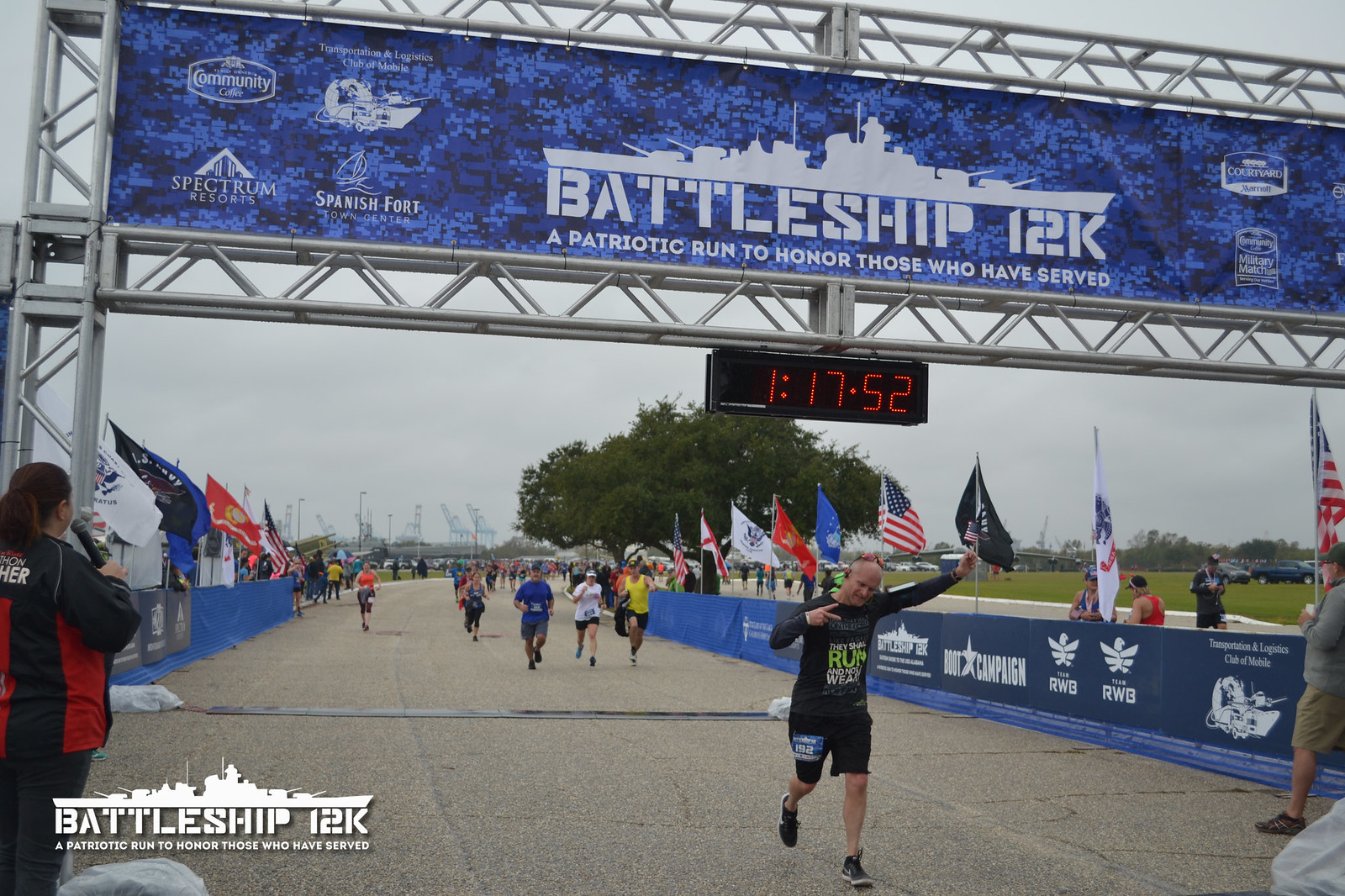In the image depicting the finish line of the Battleship 12K, a patriotic run to honor those who have served, a runner is captured just moments after completing the race with a time of 1 hour, 17 minutes, and 52 seconds. The jubilant finisher, centered at the bottom of the picture, is seen with his arms lifted in celebration. He is dressed in a black jersey with yellow print, black shorts, and black running shoes. Surrounding him, other participants can be seen approaching the finish line, some about 10 yards behind, while spectators in various colors – blue, white, and yellow – line both sides of the road.

Spanning the road is a large blue banner supported by a steel girder, bearing the outline of a battleship in white with the text "Battleship 12K" and the tagline "a patriotic run to honor those who have served." Both corners of the banner display logos from sponsors such as Spanish Fort, Spectrum Resorts, and others. Advertisements line the blue-bordered road from left to right, enhancing the celebratory atmosphere. American and military flags are prominently placed along the roadside, adding a vibrant touch to the scene. In the background, a large tree and a stretch of green field with additional trees provide a scenic backdrop to the energetic and patriotic event.